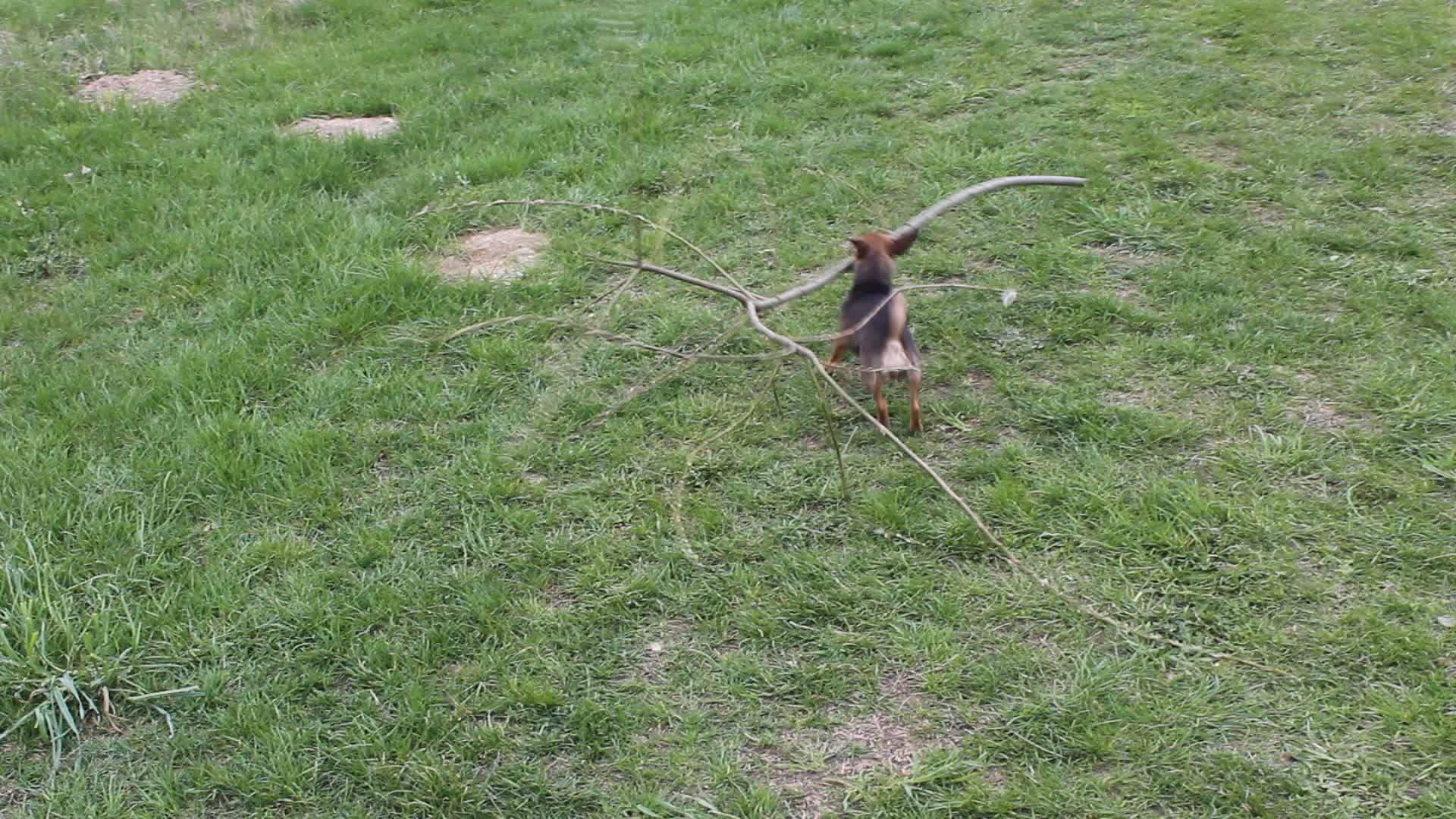This is a photograph of a small, black and brown dog, likely a chihuahua, carrying a long, irregular tree branch in its mouth. The branch is about twice the dog's length and has multiple smaller twigs sprouting from one end. The dog is walking across a yard with predominantly green grass, though some bare patches are visible where no grass is growing. The scene appears to be a typical backyard, suggested by the presence of a couple of rock steps in the top left corner. The photo is taken during the daytime, and the dog is moving away from the camera, providing a view of its back. The image is slightly blurry, emphasizing the motion of the dog as it carries its substantial stick away from the photographer.